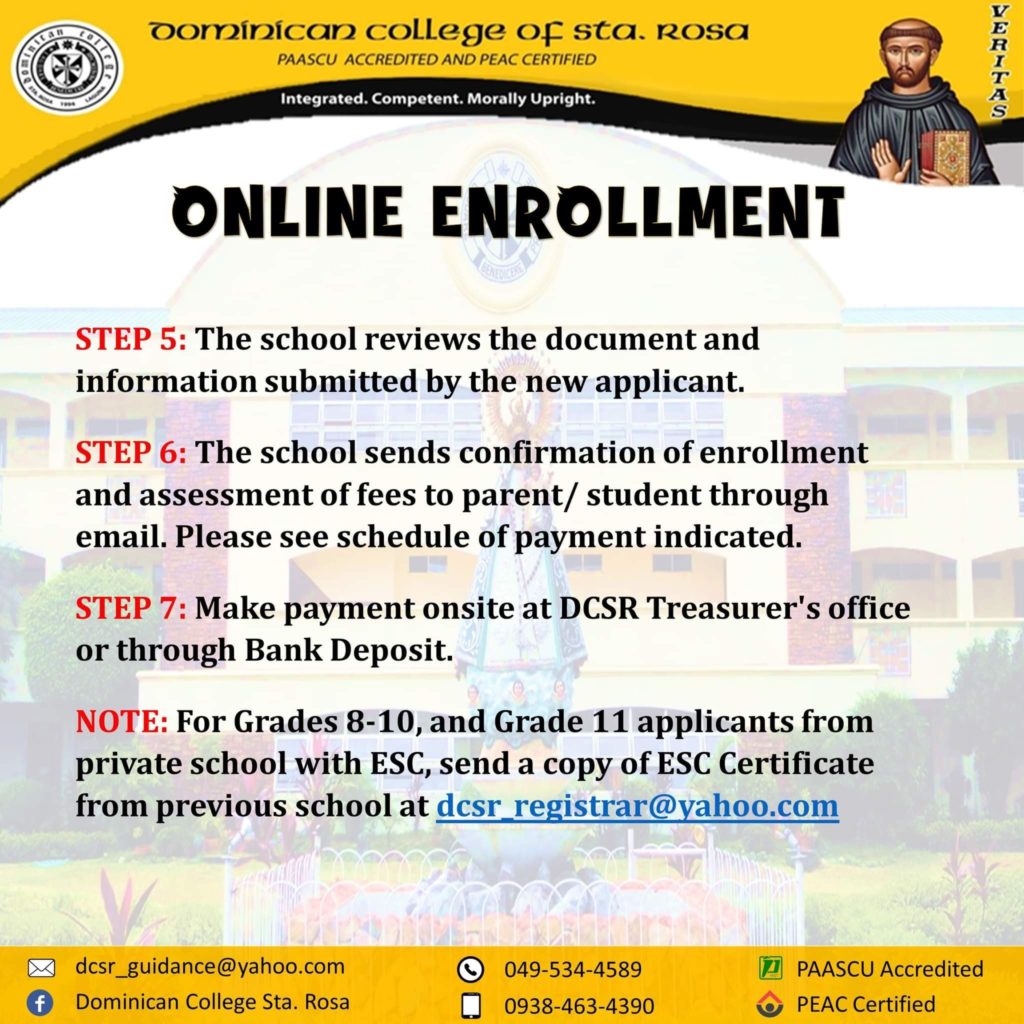The web page from Dominican College of Sta. Rosa prominently features its name at the top in lowercase black text, "Dominican College of Sta. Rosa." Directly underneath, in uppercase black text, it declares "PAASCU Accredited" and "PEAC Certified." To the right, an illustration of a monk in black robes, holding a Bible and with one hand raised, palm facing outward, appears. Beside his head, the word "Veritas" is displayed vertically in black text. This section of the page is set against a gold-yellow background accented by a curvy black ribbon below the monk.

The remaining content is superimposed over an image of the college campus. In large, bold, uppercase black text, the words "Online Enrollment" capture attention immediately. Vertical red text to the left reads "Step 5," "Step 6," and "Step 7," followed by "Note." Next to each step, in black text:

- Step 5: "The school reviews the document and information submitted by the new applicant."
- Step 6: "The school sends confirmation of enrollment and assessment of fees to parent/student through email. Please see schedule of payment indicated."

Further details continue for Step 7 and the Note. The layout and colors are carefully designed to guide prospective students and their families through the online enrollment process at Dominican College of Sta. Rosa.